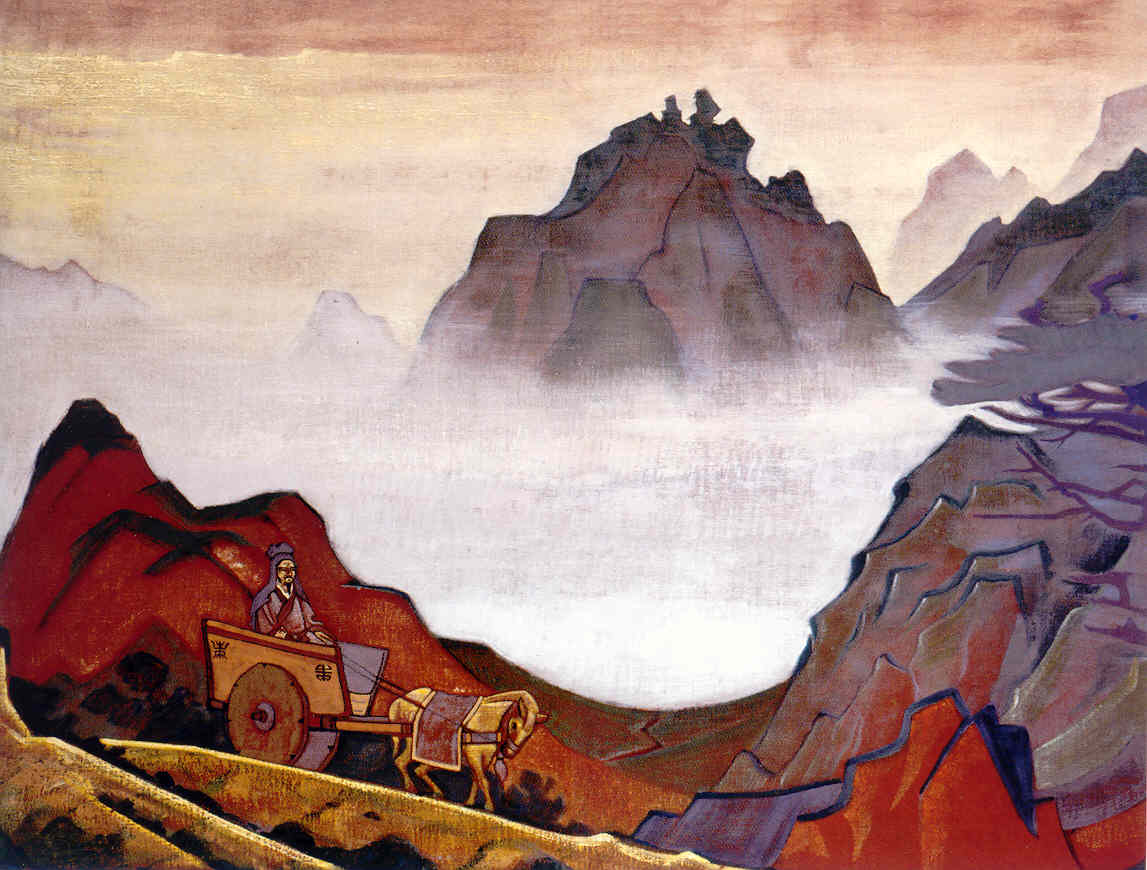The image is a richly detailed painting, seemingly medieval in style, depicting a dramatic mountain landscape at sunset. The scene centers on an Asian man in a horse-drawn cart, positioned in the foreground. The man is dressed in a long blue and red robe with a red scarf on his head, and the horse pulling the cart is golden with a blanket draped over its back. 

The mountains are rendered in layers, with vibrant reds, blacks, purples, and browns in the foreground, and softer, more distant peaks of reds and blacks, interspersed with fog. The sunset casts a warm orange and yellow glow across the sky, adding to the painting's ethereal quality. The structural and geometrical rocky mountains dominate the middle and background, gradually fading into the foggy valley below, creating a sense of depth and vastness.